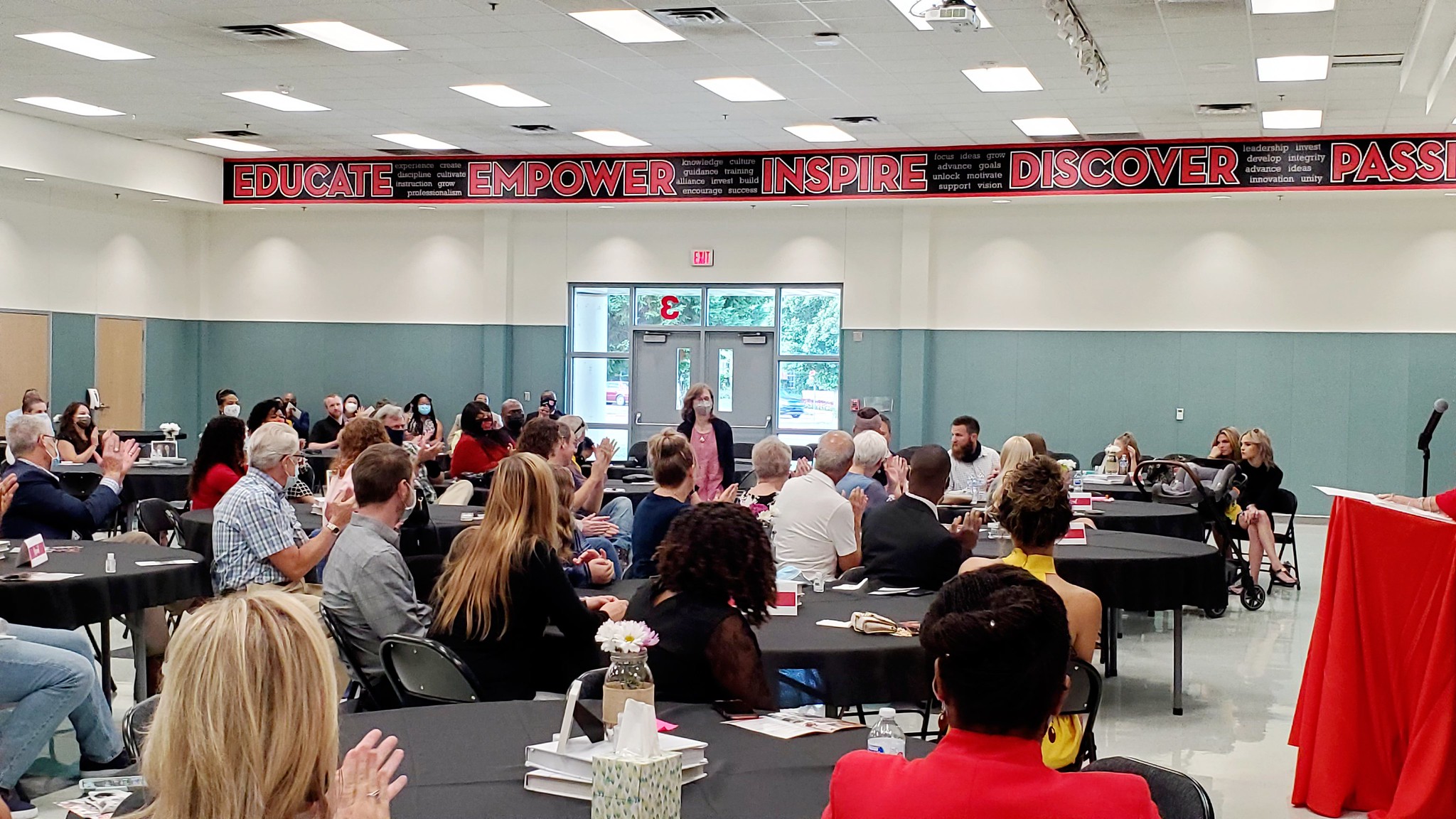The image depicts a large group of adults attending an education or inspirational conference in a well-lit meeting room, likely a community center or hall. The attendees are seated around round tables draped with black tablecloths, all focused on a woman standing at the center front of the room. She is wearing a pink shirt under a black jacket, has brown hair, and is wearing a gray mask. She appears to be speaking or asking a question, as the audience is clapping. 

The room features a prominent black banner across the back wall with bold red text that reads "Educate, Empower, Inspire, Discover," and partially visible text starting with “P-A-S-S.” The banner is set against a background where the top part of the wall is white and the bottom part is a light green. Above the double swinging doors at the center of the back wall, there is a backwards number three and an exit sign. Fluorescent rectangular lights illuminate the white ceiling and cast shadows on the upper walls.

On the right side of the image, a podium draped in a red cloth stands with a black microphone and a white paper on top, where a hand rests, suggesting the person previously speaking is now seated. The overall scene captures the engaged ambiance of a formal event dedicated to education and inspiration.